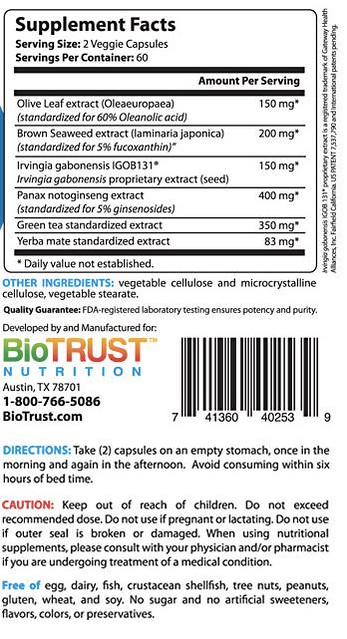Here's a descriptive caption:

"This image showcases a nutrition label from a Biotrust Nutrition product. The label itself does not specify the product name but lists various ingredients including olive leaf extract, brown seaweed extract, verbena, gabonensis, panax ginseng, green tea, and yerba mate. The label features a barcode and direction instructions beneath it. The text on the label is predominantly black on a white background, with 'Biotrust' highlighted in green and orange letters and 'Nutrition' in blue letters, adding a touch of brand-specific color to the packaging."